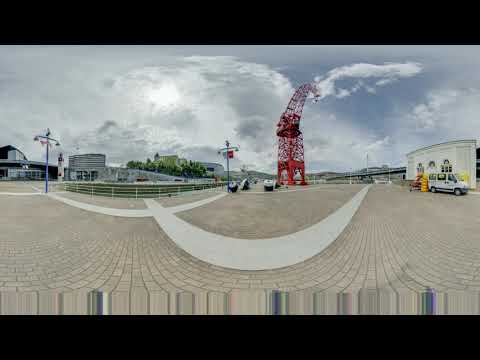The panoramic photograph captures an outdoor setting with a light-colored brick pavement showcasing a slightly distorted and curved perspective, typical of a wide-angle lens. Dominating the off-center of the image is a tall red structure, likely a crane, juxtaposed against a cloudy daytime sky that allows partial sunlight to filter through. A white van is parked on the right side next to a white building or structure, in front of which appears to be yellow items, perhaps cargo being handled. Further right in the background, a bridge is visible. The left side features a red and white building with a curved second story, adjacent to a small fenced-in area with vegetation and smaller buildings. The scene also includes poles that could be streetlights and several multi-story buildings enveloped by trees in the distance, adding depth to the landscape. The image's lower section is slightly blurred and pixelated, adding a unique effect to this serene yet industrious outdoor snapshot.